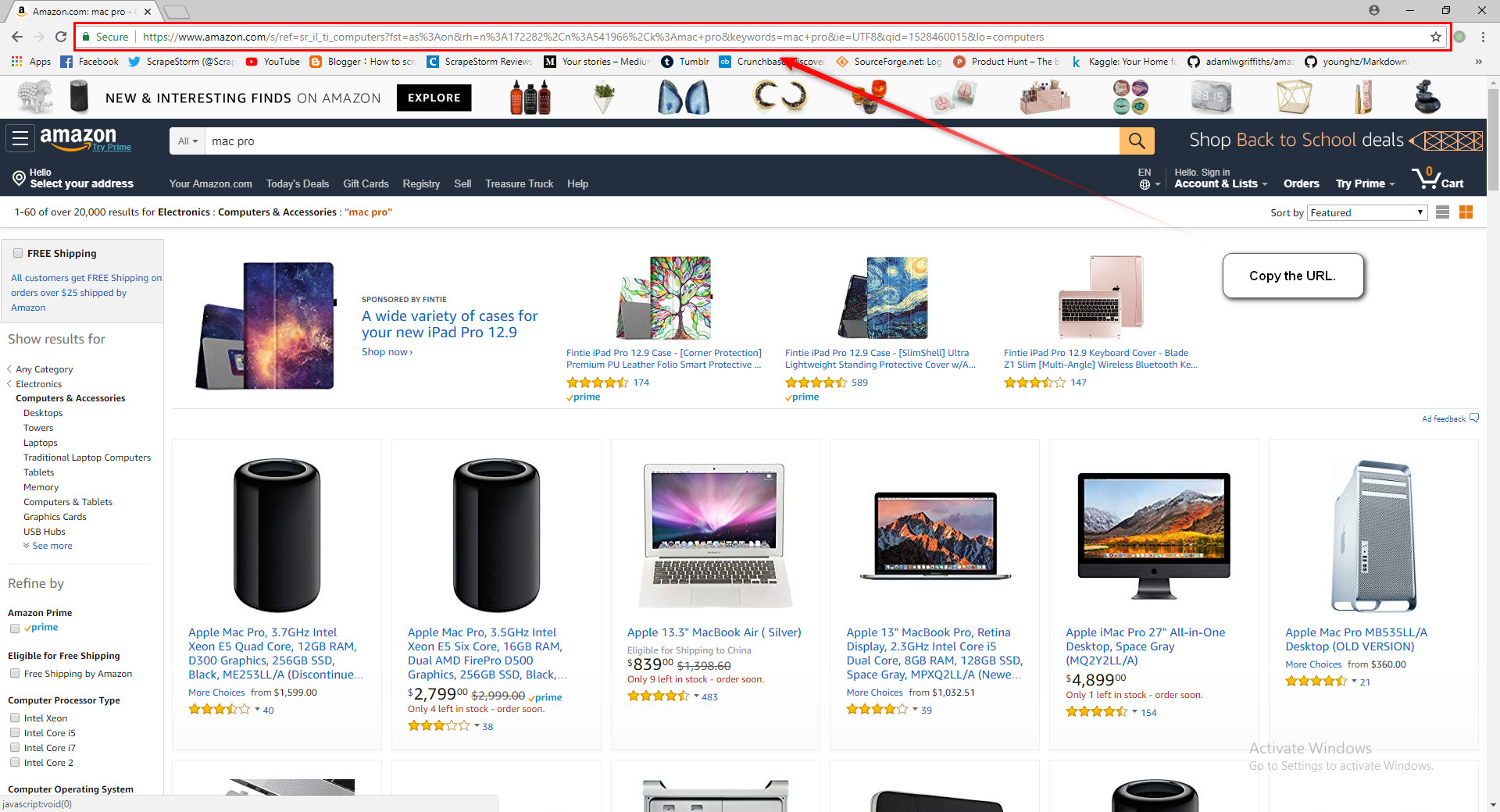The image is a screenshot from the Amazon website. In the upper-left corner, the Amazon logo is prominently displayed in white. Beside it, to the right, is a search bar. Above this search bar, the web address bar is outlined in red, drawing attention with a red arrow pointing towards it.

Beneath the address bar sits another search bar. In the left-hand corner of the page, there are white flowers and an Alexa device, accompanied by the text "New and interesting finds on Amazon" written in black. Next to this, within a black box containing the word "Explore" in white text, a variety of items are arranged prominently, including shampoo bottles, flowers, two blue rocks, and semi-hoop earrings. 

Further to the right, the image features an assortment of cups, followed by pictures of flowers, a basket, and four stones arranged in a square. Next in line is a white basket, a gold basket, a colorful item that appears to be a bookend, and a pair of black goggles.

Lower on the page, the Amazon logo appears again alongside another white search bar. Below this section, there are several images of products starting with what looks like a Kindle cover. To the right of this cover is an advertisement suggesting a variety of cases for the new iPad Pro 2.9, depicted in blue. Adjacent to this are three more iPad cases: one featuring a solar system pattern, another showcasing a brown tree with pink flowers, one displaying Van Gogh’s famous painting in shades of blue, and one in plain pink.

Further down, there are two images of Alexa devices side by side. To the right of these are images of a white MacBook Pro, a black MacBook Pro, and a black desktop monitor. Lastly, a stainless steel case described as an old version desktop case is displayed to the far right.